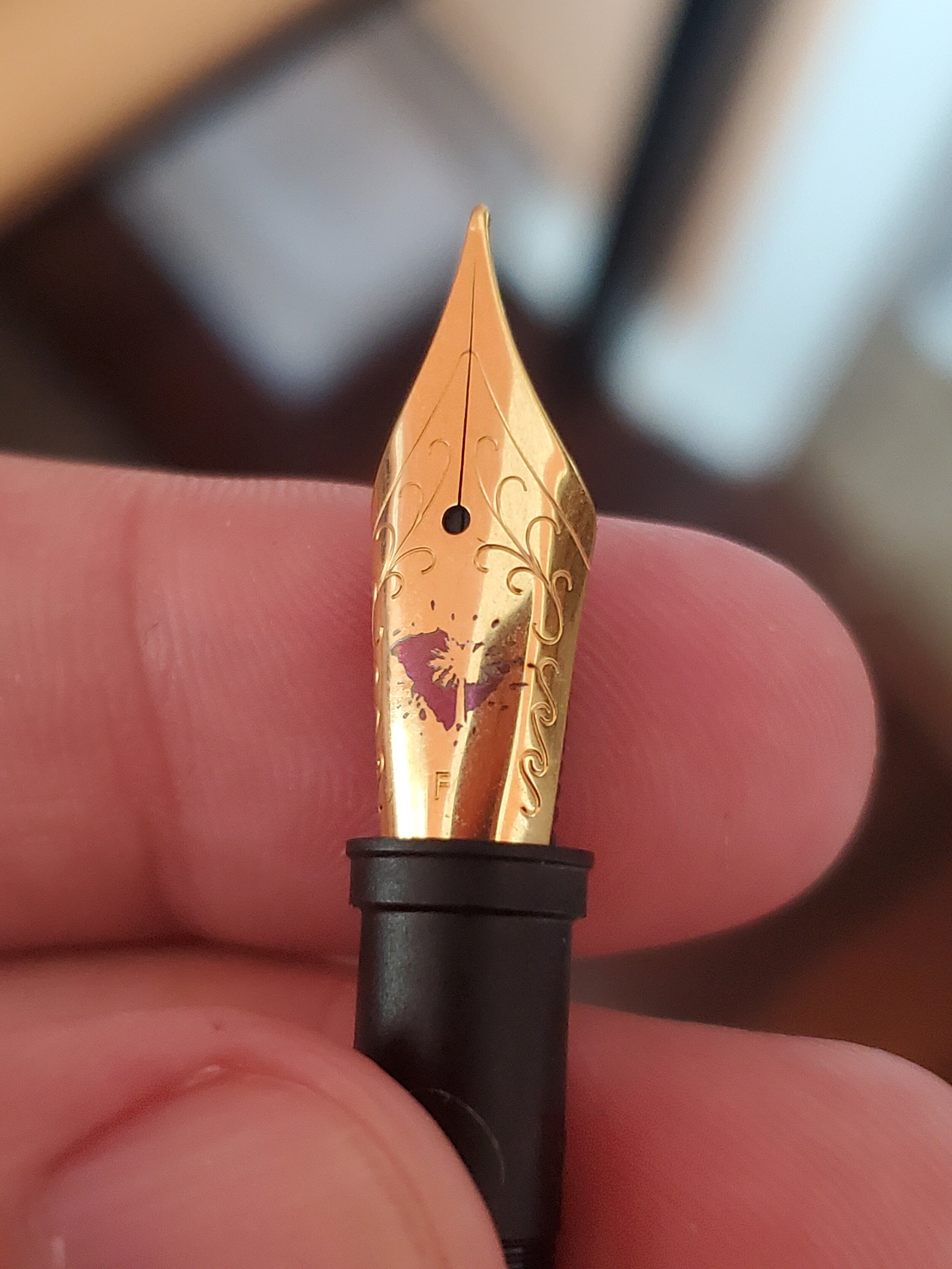In the image, a photorealistic close-up captures the intricate details of a gold fountain pen nib held by a white male hand. The hand, positioned from the left, shows only the upper joints of the thumb, index, and middle fingers, which grip the black base of the pen. The nib, adorned with ornate scroll and vine designs, also features an "F" inscribed on it, accompanied by a small red blotch. The black handle of the pen resembles a flower pot. The background is intentionally blurred, revealing an abstract mix of pale tan triangles and indistinct squares and rectangles in lighter gray and brown hues, potentially depicting paper and architectural elements. The overall focus clearly emphasizes the elegance of the gold nib and the craftsmanship of the pen.